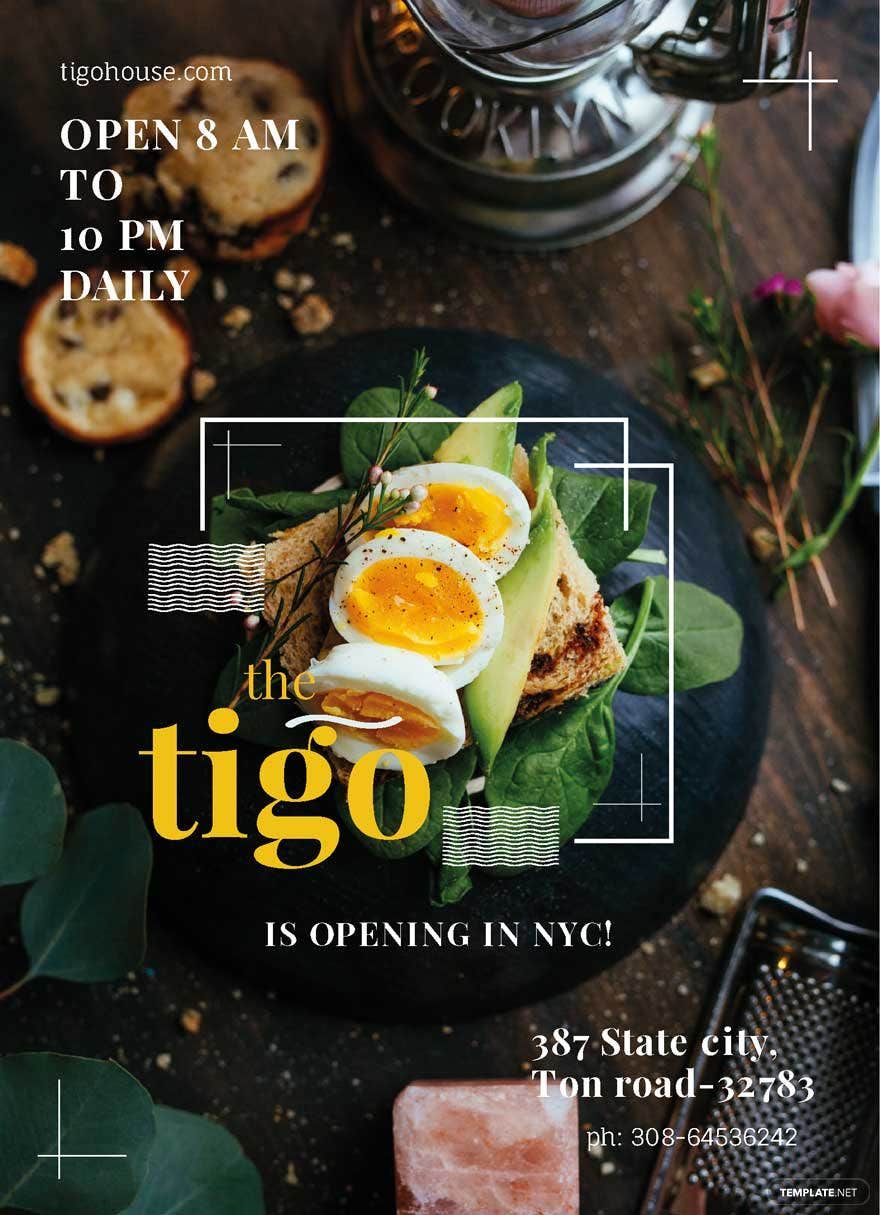This image appears to be a magazine cover or advertisement for a new restaurant. In the top left corner, the URL "teagohouse.com" is displayed in white text. The background features an elegant, modern table setting on a dark wood surface. 

On the top left of the table, there is a small office space adorned with cookies. At the center of the table, there's a mouthwatering dish of medium-boiled eggs with a sprinkle of pepper and herbs, placed on top of avocado toast. This delicious arrangement is framed by two white half-borders and some wavy designs just below the eggs on the left side.

In the middle of the image, the restaurant's name, "teagoh" is prominently displayed in lowercase yellow letters with a wavy white line accentuating the G. Below the restaurant name, there is white text announcing the restaurant's opening in "New York City, NYC!" 

Additionally, an address and phone number are provided in white text at the bottom right corner of the image.